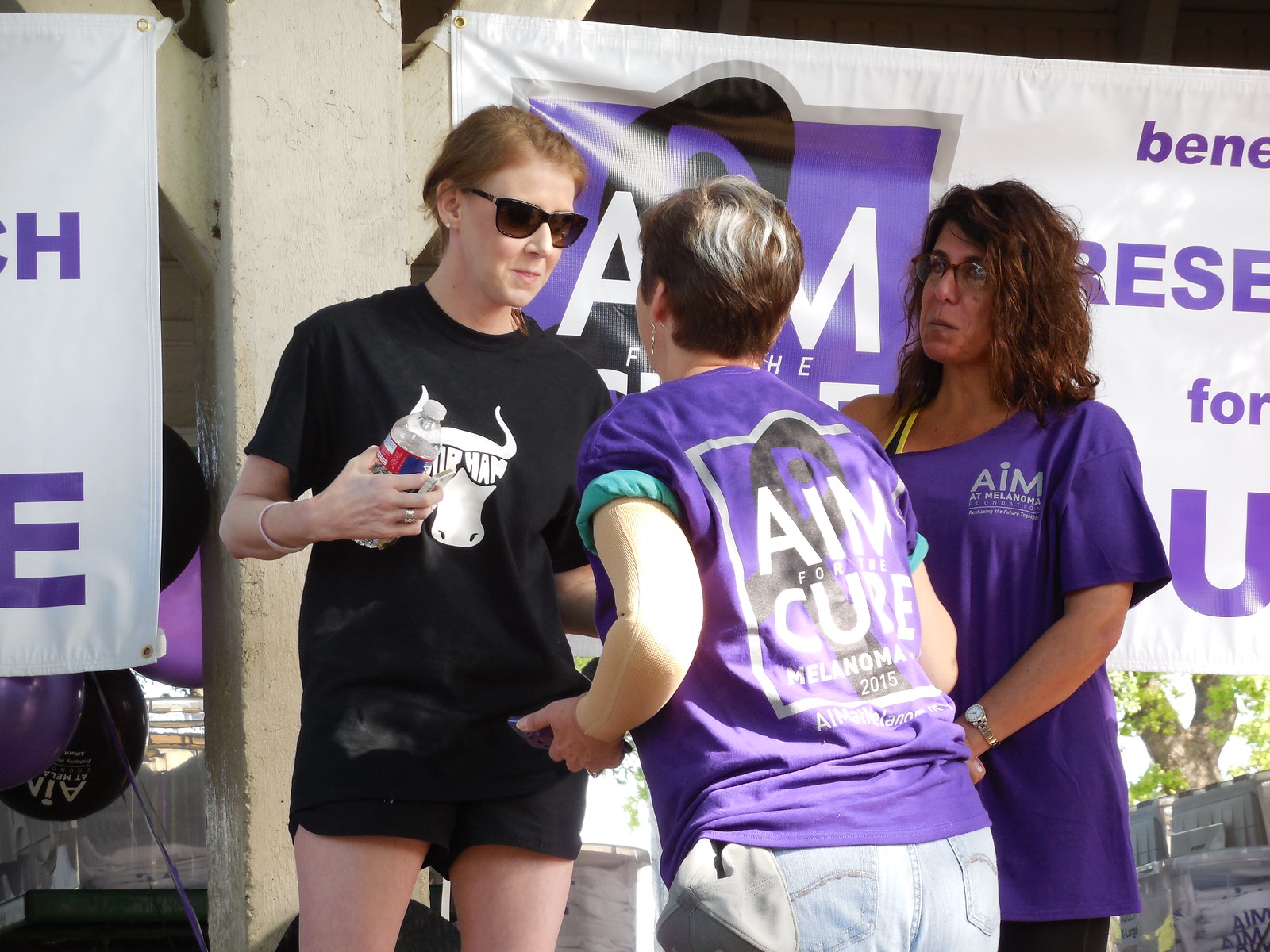This outdoor photographic image captures a scene of three women at a fundraising event. The primary focus is on a woman with red hair styled in a small ponytail, who is wearing dark sunglasses, a black T-shirt featuring a graphic of a cow with sunglasses within the letters "I-P-H-A-M," and very short black shorts. She is accessorized with a bracelet and a ring and holds a water bottle in her left hand. She appears engaged in a conversation with another woman, who is turned away from the camera. This second woman has short, multicolored hair—possibly black with blonde or gray tints—and is wearing purple lymphedema sleeves. Her purple T-shirt reads, “Aim for the Cure, Melanoma 2015” and “Aim Melanoma” underneath. The third woman, standing to the right and observing, has shoulder-length brown hair, glasses, and is also clad in a purple T-shirt emblazoned with “Aim at Melanoma Foundation” and “Reshaping the Future Together.” The background features a wall with a partially visible banner stating, “Aim for the Cure,” and other text obscured from view. Additionally, a partially visible poster with the letters "H" and "E," a structural pole, and a tree are in the backdrop, along with purple balloons contributing to the festive atmosphere.